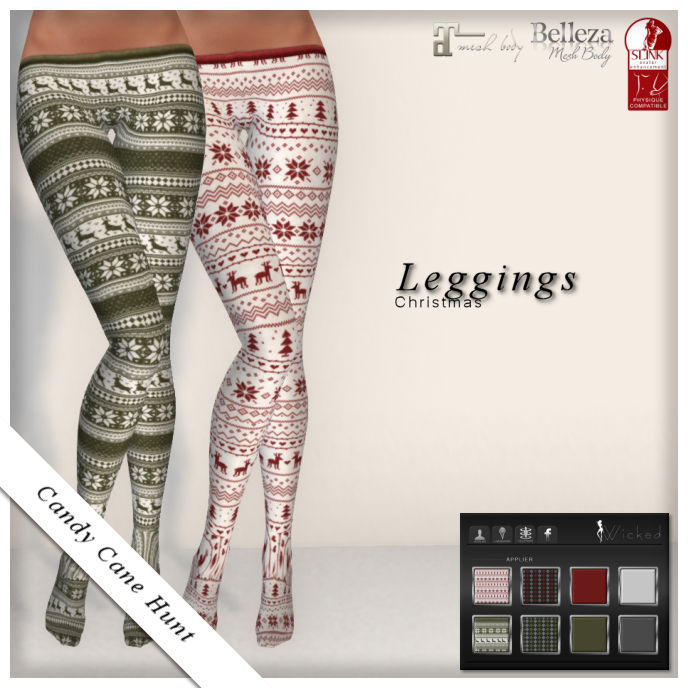The advertisement features a beige background with holiday-themed leggings prominently displayed on the left side. The image shows two women from the waist down, wearing festive leggings that appear to be a classic Christmas pattern you'd find in flannel. The pair on the left is a pine green and cream color with snowflakes, stripes, and reindeer designs. The pair on the right is brighter white, adorned with red trees, red snowflakes, and red reindeer standing next to hearts. Both pairs of leggings extend to cover the ankles, with their toes hidden.

A diagonal banner near the bottom of the image, also a little upwards from it, reads "Candy Cane Hunt" in green. Above this banner, centrally located, is the text "Christmas Leggings." In the bottom part of the advertisement, a color chart is visible, showing the available different patterns including white, red, and other variations. The upper right corner includes logos for mesh body brands like Belize and Slink. The leggings, clear from the descriptions, are digitally rendered to highlight their festive patterns.